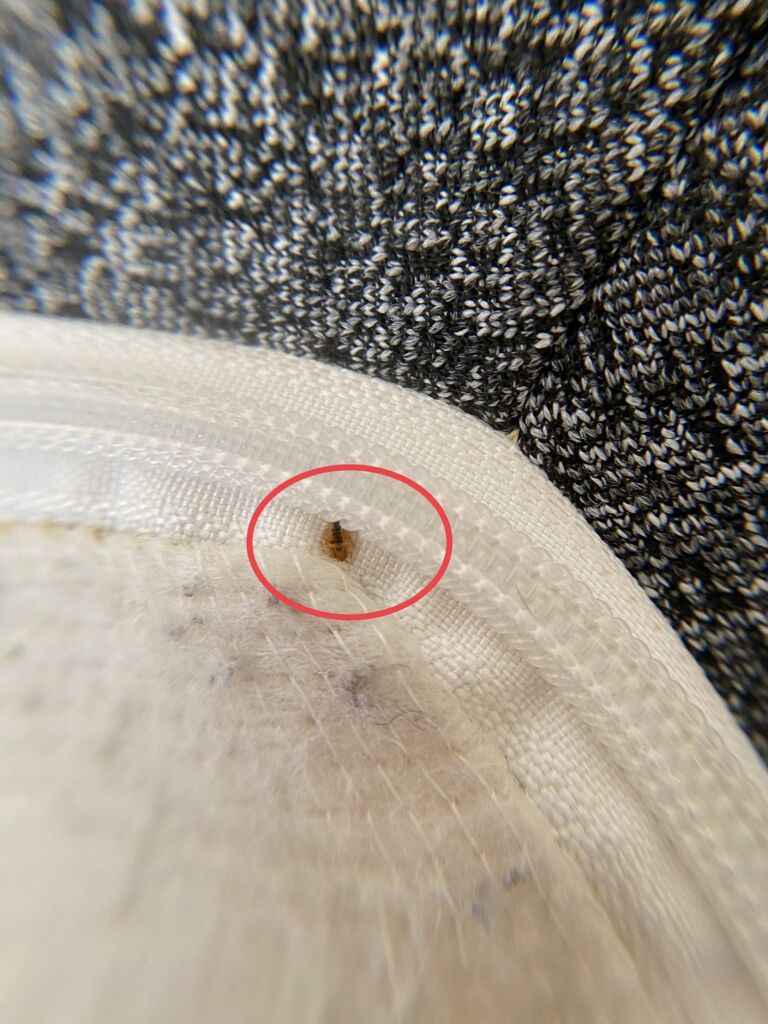The image is a close-up of a dirty, frayed mattress corner, specifically focusing on a single insect that is likely a bed bug. The bug, encircled in red for clear identification, has a light orange body with a distinctive black streak down the middle of its thorax. The mattress, covered with a white fitted sheet that is pulled tightly over it, appears soiled and aged. The upper part of the frame shows black and white fabric, slightly out of focus, with some dark material and fur mixing into the scene. This insect is conspicuously positioned within the crease of the mattress, emphasizing concerns about bed bugs in this context.